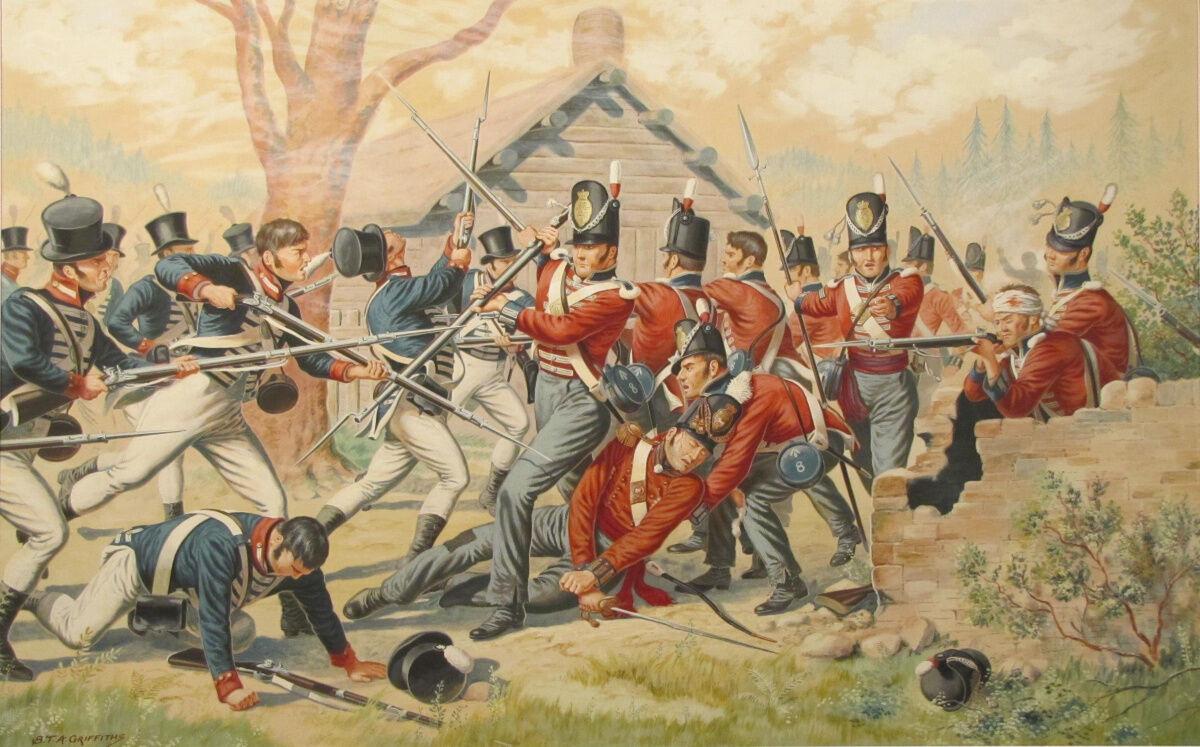This detailed artwork, likely a drawing or painting, depicts a Revolutionary War battle scene set outdoors. The sky is yellow with white clouds, suggesting either dawn or dusk, with smoke lingering in the air, indicative of gunfire. The battleground is predominantly brown earth with patches of green grass. A brown log cabin house with a chimney stands in the background, adjacent to a leafless brown tree that extends off the top of the image. In the bottom left corner, the artist's signature "S.T.A. Griffiths" is visible in brownish-black letters.

The right side of the image features soldiers wearing distinct red uniforms with black pants, black shoes, tall hats adorned with a gold badge, and white-and-red feathers. A brick wall with missing chunks and a small shrub partially obscures some of these red-uniformed soldiers. One soldier, wearing a white headband, aims his rifle with a silver bayonet from behind the wall. Another red-uniformed man assists a fallen comrade who has been hit and is lying on the ground.

Conversely, the left side shows blue-uniformed soldiers with black top hats, white trim, white pants, and black boots. In the foreground, a blue-uniformed soldier stands, poised to strike with his bayonet at an opponent in red who is on his hands and knees, his gun lying under him. The scene also includes more soldiers from both sides engaged in fierce combat, wielding long spear-like bayonets. Amidst the chaos, a man on his knees is being pulled back by another soldier grabbing him under the armpits.

Overall, the image captures the intensity and brutality of the battle, with detailed uniforms, weaponry, and the chaotic environment vividly rendered.